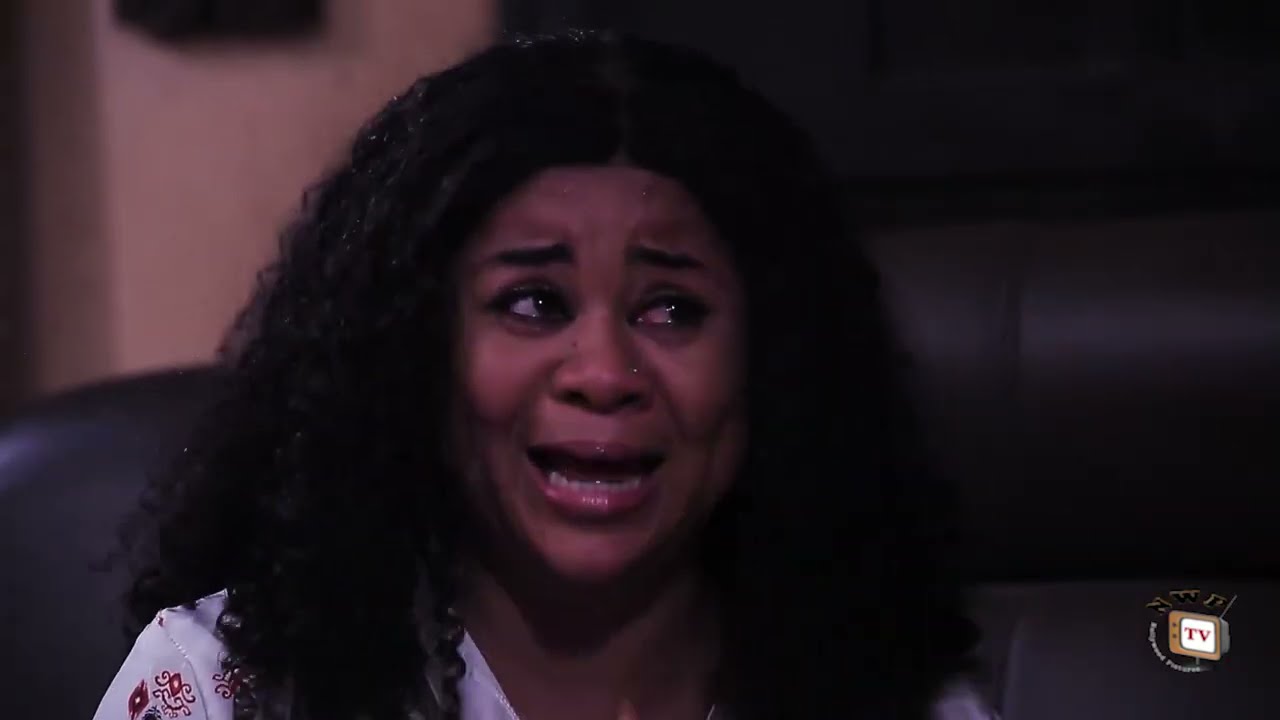The image features a close-up of a black woman with a dark complexion, sitting on a dark couch—either black or dark brown. She has thick, tightly curled black hair cascading to her shoulders. She wears a floral-patterned white shirt with a V-shaped collar and possibly some frilly lines and red diamond shapes. The expression on her face is one of deep distress; her teary eyes glisten as she looks to her left, her eyebrows furrowed, and her mouth opens in a pained grimace, revealing her lower teeth. The background consists of a beige wall, indicating an indoor setting. In the bottom right corner of the image, a small TV logo with the word "TV" adds a hint that this could be a still from a television program. The overall atmosphere of the image is somber, emphasizing her emotional turmoil and the intense moment of sorrow or fear she is experiencing.